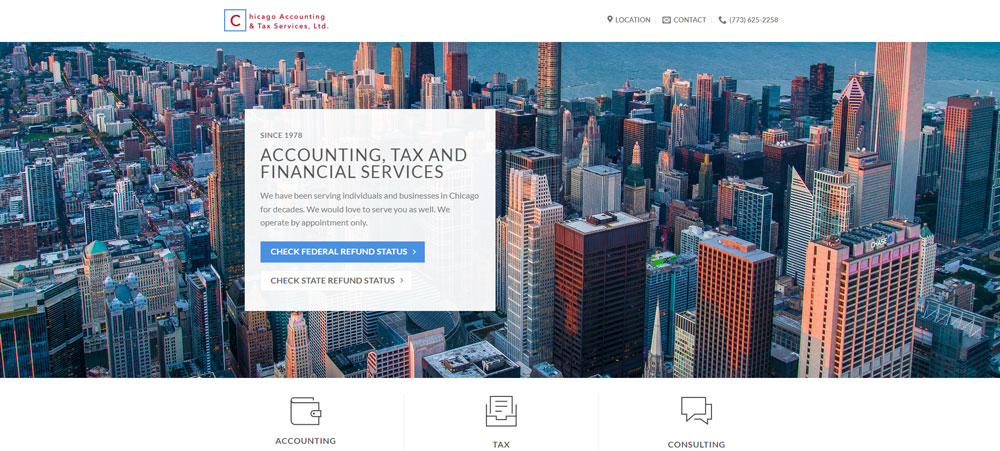**Caption:**

Advertisement for Chicago Accounting and Tax Services, LTD

The top of the advertisement prominently features the company's name, "Chicago Accounting and Tax Services, LTD," with the first letter "C" uniquely enclosed in a box. Adjacent to this, a GPS icon indicates location details, followed by a contact icon and a phone number for direct reach. 

Dominating the central portion of the screen is a striking aerial view of Chicago showcasing its iconic tall buildings and dense urban landscape. This image serves to localize and contextualize the services offered by the company within the bustling city.

Beneath this imagery, a text box reads, "Since 1978, Accounting, Tax, and Financial Services. We have been serving individuals and businesses in Chicago for decades. We would love to serve you as well. We operate by appointment only." This statement emphasizes the company's long-standing history and commitment to personalized service.

Towards the bottom, the advertisement features interactive elements: a blue clickable box labeled "Check Federal Refund Status" and a white clickable box labeled "Check State Refund Status." These boxes are designed to provide quick access to tax refund information.

Finally, three icons are displayed representing the company's core services: accounting, tax, and consulting, though it’s unclear if these icons are clickable. This visual layout succinctly encapsulates the comprehensive range of professional services offered by the firm.